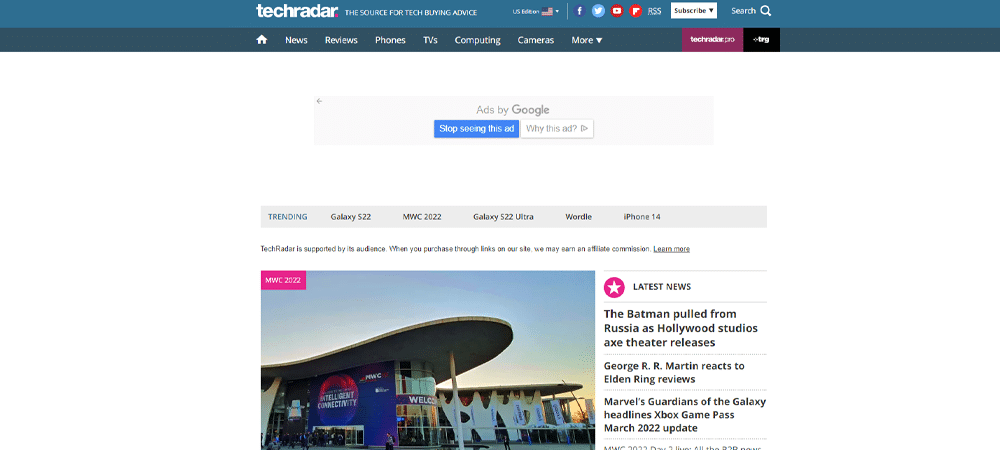The image is a screenshot of the TechRadar website viewed on a laptop. The website features a predominantly white background. At the top, there is a blue banner displaying the TechRadar logo in white lettering, along with a search button. Just below this banner, there's a darker navigation bar with white text that offers links to various sections such as News, Reviews, Phones, TVs, Computing, Cameras, and more.

Immediately beneath the navigation bar, there's a "Ads by Google" label followed by an advertisement. The ad features a photograph of a theater and has a headline that reads, "The Batman Pulled From Russia As Hollywood Studios Acts Theater Releases." 

Further down, the webpage contains various navigational buttons for browsing through different trending topics, galleries, and other website sections, including a specific page dedicated to the iPhone 14.